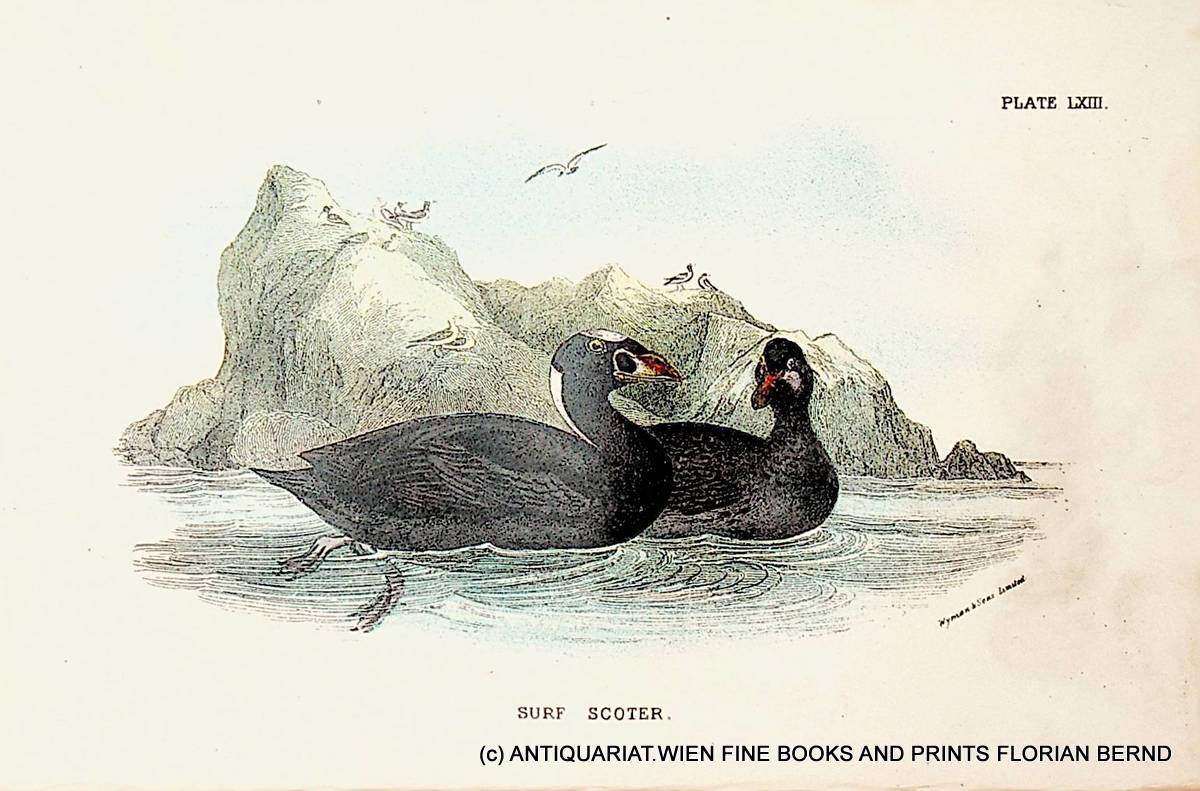This detailed illustration, likely from the 18th or 19th century, features two ducks—known as surf scoters—swimming in tandem on a body of water. The art, rendered in ink and colored using mediums such as colored pencils or watercolors, depicts the duck closest to the viewer in a full profile with both of its feet visible paddling beneath the water, while the other duck, slightly more oriented towards the viewer, has no visible feet. The ripples in the water are prominently illustrated, adding a sense of movement. In the background, there's a prominent outcropping of rock adorned with several seagulls, some perched and one flying away. The image is framed as a plate from a book or similar publication, identified as plate LXIII in the upper right corner. At the bottom, non-bold text details the title "Surf Scoter" and attribution to "Antiquariate, Wien, Fine Books and Prints, Florian." The overall color palette is muted, reinforcing the illustration's antiquarian aesthetic.